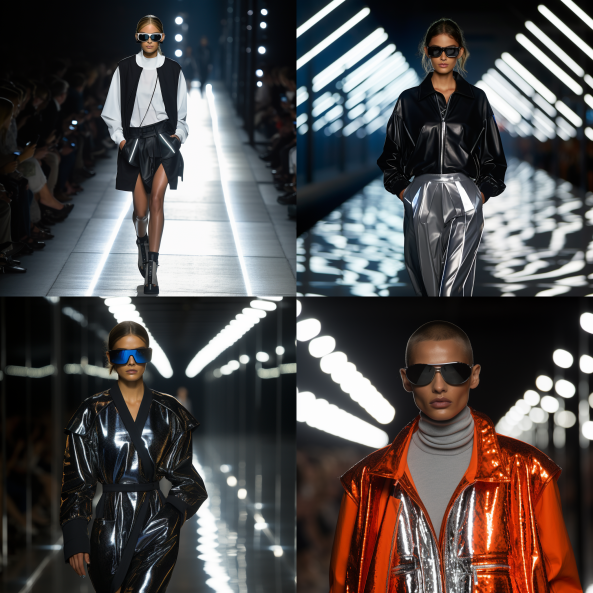The image is a collage of four panels, each featuring a different runway model in a high-fashion show. 

In the top left panel, a white woman with brunette hair pulled back is seen striding down a runway illuminated in white. She wears futuristic sunglasses, a white sweater under a black vest, paired with tights and boots. The audience lines both sides of the runway, which is primarily visible through its bright lighting.

The top right panel displays the same woman, her hair now down, dressed in a black leather coat and shimmering platinum silver pants. She has her hands casually placed in her pockets and dons black sunglasses. The runway remains brightly lit, with rows of lights enhancing the background.

The bottom left panel shows the same model again, this time wearing larger, blue-tinted sunglasses and a long, shimmering black coat. The fully lit runway and background lights offer a consistent backdrop.

In the bottom right panel, a male model takes the stage. He wears black sunglasses and a shimmering orange and silver coat over a gray turtleneck. His hair is short, almost shaved. Similar to the other panels, background lights illuminate the scene, though the runway is obscured by his figure.

All models share a coordinated aesthetic with their futuristic and shimmering attire, set against a backdrop of a well-lit runway and enthusiastic, yet shadowed, spectators.